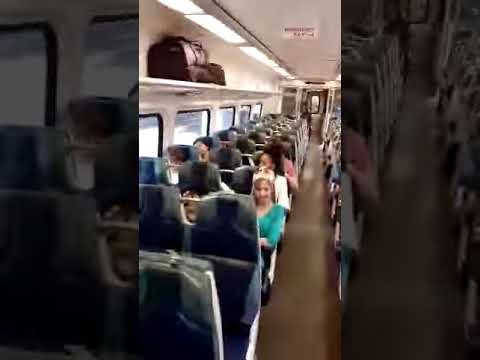The image depicts the interior of a train, characterized by a long aisle flanked by rows of blue seats on either side. The train's flooring appears tan or brown, while its interior walls and ceiling are white. Large windows line the left side, and above them, a shelf running parallel to the aisle holds a few pieces of luggage, with one prominently brown bag to the left. The ceiling is outfitted with long fluorescent lights and features an illegible sign, possibly indicating an emergency exit. Among the passengers, a woman in a teal-colored blouse is most prominent, followed by a second woman in a white blouse, and a third person in a pink or red shirt can also be faintly seen farther back. The image is somewhat blurry and is encapsulated by wide borders on the left and right, created by enlarging and blurring elements from the main picture to frame the scene. At the far end of the aisle is the door leading to the next train car.